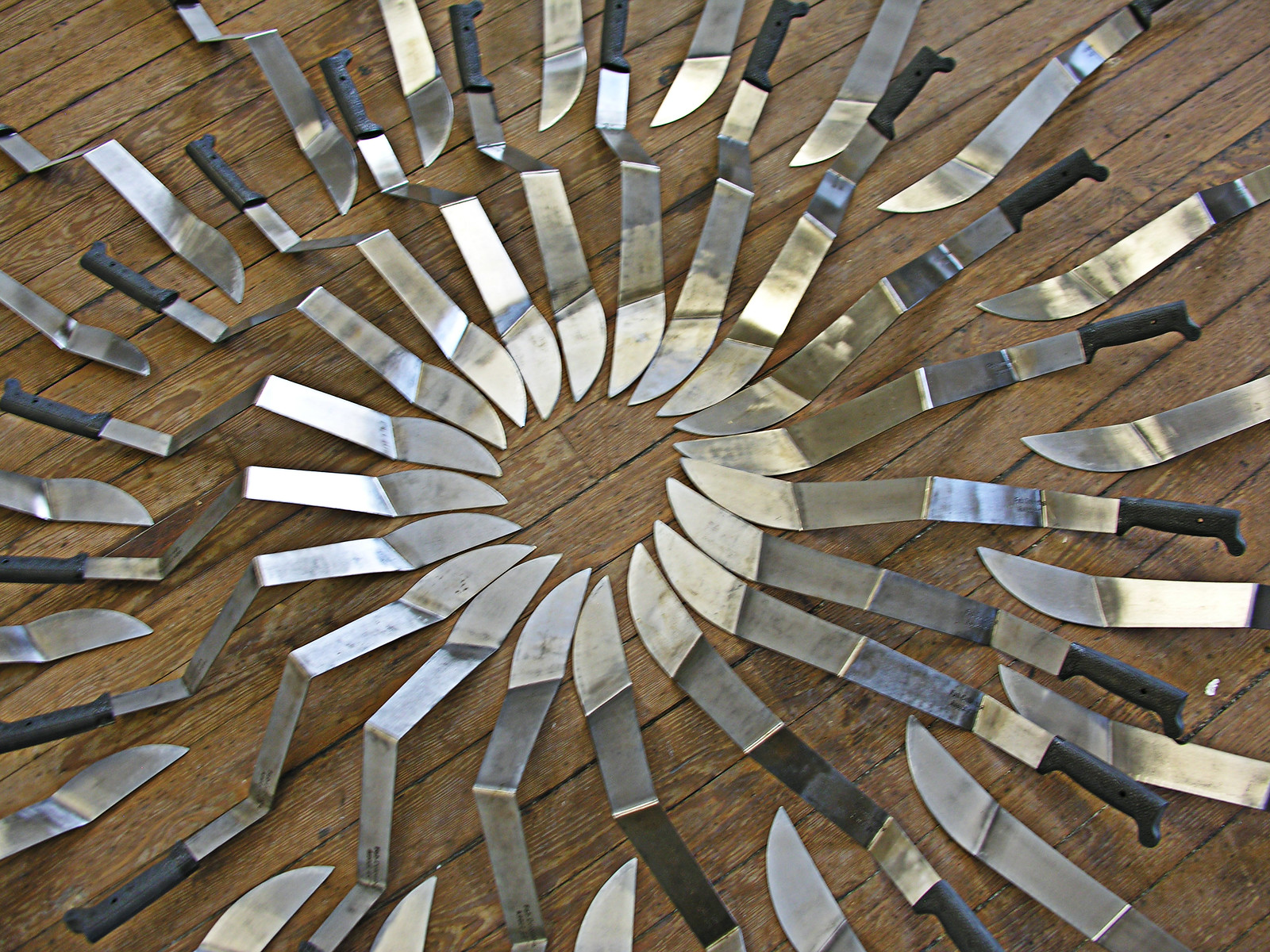The image showcases an intricate art installation composed of numerous machete-like knives. Each knife features a long, silver blade—approximately 18 inches in length—bent at multiple sharp angles: down, up, down, and up again, creating a ripple effect. These blades are meticulously arranged in a tight, circular formation with their tips meeting precisely at the center, resembling the bloom of a flower or the teeth of a saw. The knives, all identical with black handles, extend outward from the center, forming a geometric pattern. Secondary blades fill the gaps between the handles, enhancing the density of the array. The entire installation rests on an aged, well-worn wooden floor, emphasizing the contrast between the cold, metallic blades and the warm, grainy wood. This striking setup evokes a sense of abstract, almost surreal beauty and symmetry.